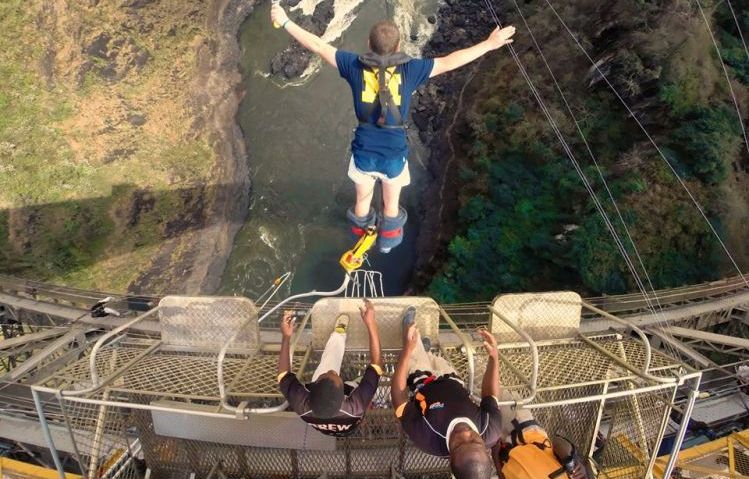The image captures a thrilling moment of a bungee jump from a top-down perspective. A person dressed in a navy blue shirt adorned with a yellow Michigan "M" logo and shorts is in mid-air, arms outstretched. Their short brown hair flutters as they plummet towards a dark green body of water below. Gray straps are securely fastened around their ankles, connecting them to a white bungee cord. The jump platform is visible beneath them, with two instructors dressed in black t-shirts and white pants standing on its white surface, having just assisted in the jump. On the left side of the image, there is a lush green field punctuated with patches of brown, while the right side reveals a densely treed area boasting various shades of green. Power lines stretch across the scene, and a distinct grate structure on top of the bridge marks the sophisticated setup for the bungee jump. The entire scene encapsulates the contrast between the mechanical setup of the bungee jump and the serene, verdant landscape below.